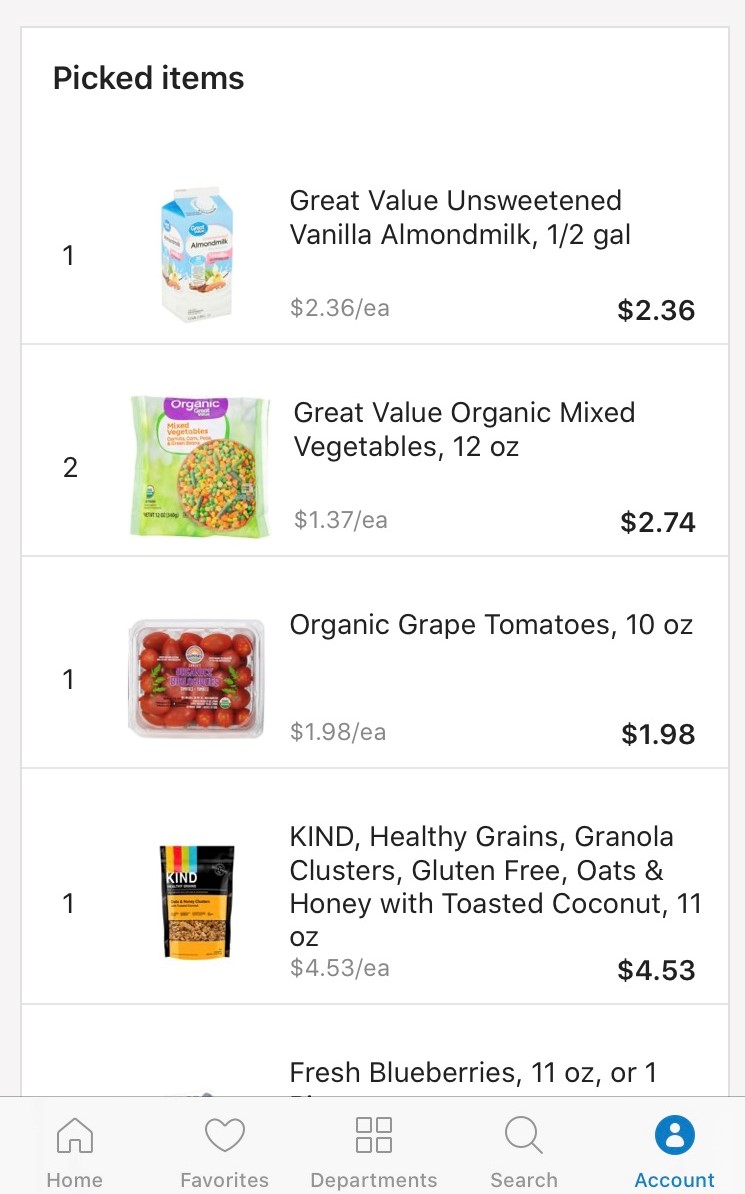The image features a light blue background with a large white box labeled "Picked Items." Within this main box, there are four individual white boxes, each outlined in light blue, containing details about different grocery products:

1. **Great Value Unsweetened Vanilla Almond Milk** - Half a gallon, priced at $2.36 each.
2. **Great Value Organic Mixed Vegetables** - 12 ounces, priced at $2.74 each.
3. **Organic Grape Tomatoes** - 10 ounces, priced at $1.98 each.
4. **Kind Healthy Grains Granola Clusters (Gluten-Free, Oats and Honey with Toasted Coconut)** - 11 ounces, priced at $4.53 each.

Additionally, there is a listing for **Fresh Blueberries** - 11 ounces. Each product listing is set within its individual white box surrounded by a light blue outline.

At the bottom of the image, there is a light blue strip containing navigation options labeled "Home," "Favorites," "Departments," "Search," and "Account." The overall layout is clean and organized, with light blue elements providing a cohesive design.